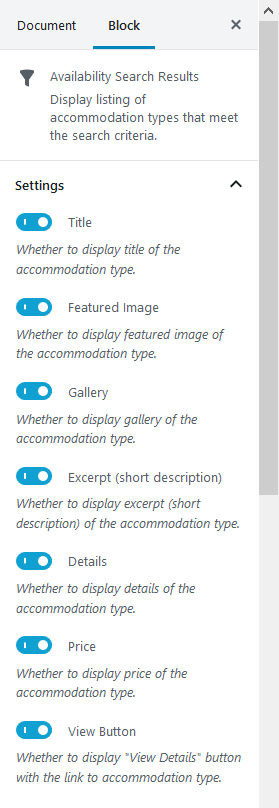This screenshot captures a detailed settings interface for an application, likely related to managing accommodation listings. 

- **Header Section:** At the upper left corner, the label "Document" is displayed. In the center top area, the word "Block" is highlighted with a blue underline. To the upper right, there's an exit arrow icon. A vertical scroll bar is present on the right side, implying that more options are viewable upon scrolling.

- **Main Settings Panel (Left Side):**
  - **Availability:** This section appears to manage the search results for accommodations. Below "Availability," there is a series of listing display options.
  - **Display Listing Options:**
    - **Title:** A toggle switch is shown in the "on" position, indicating the configuration to display titles of the accommodation types.
    - **Featured Image:** Another toggle switch is on, set to show the featured image of the accommodation type.
    - **Gallery:** This toggle switch is also on, allowing the display of a gallery for the accommodation type.
    - **Excerpt:** Set to display short descriptions, as indicated by an active toggle switch.
    - **Details:** The next toggle switch is on, set to show detailed information about the accommodation type.
    - **Price:** The active toggle switch indicates that prices for each accommodation type will be displayed.
    - **View Button:** The final toggle switch is on, enabling the view details button for users to see more information about the accommodation types.

The panel is well-organized, providing granular control over which information about the accommodations is displayed to users. Each toggle switch represents a different element that can be configured, ensuring that the display settings are customizable to meet specific needs.